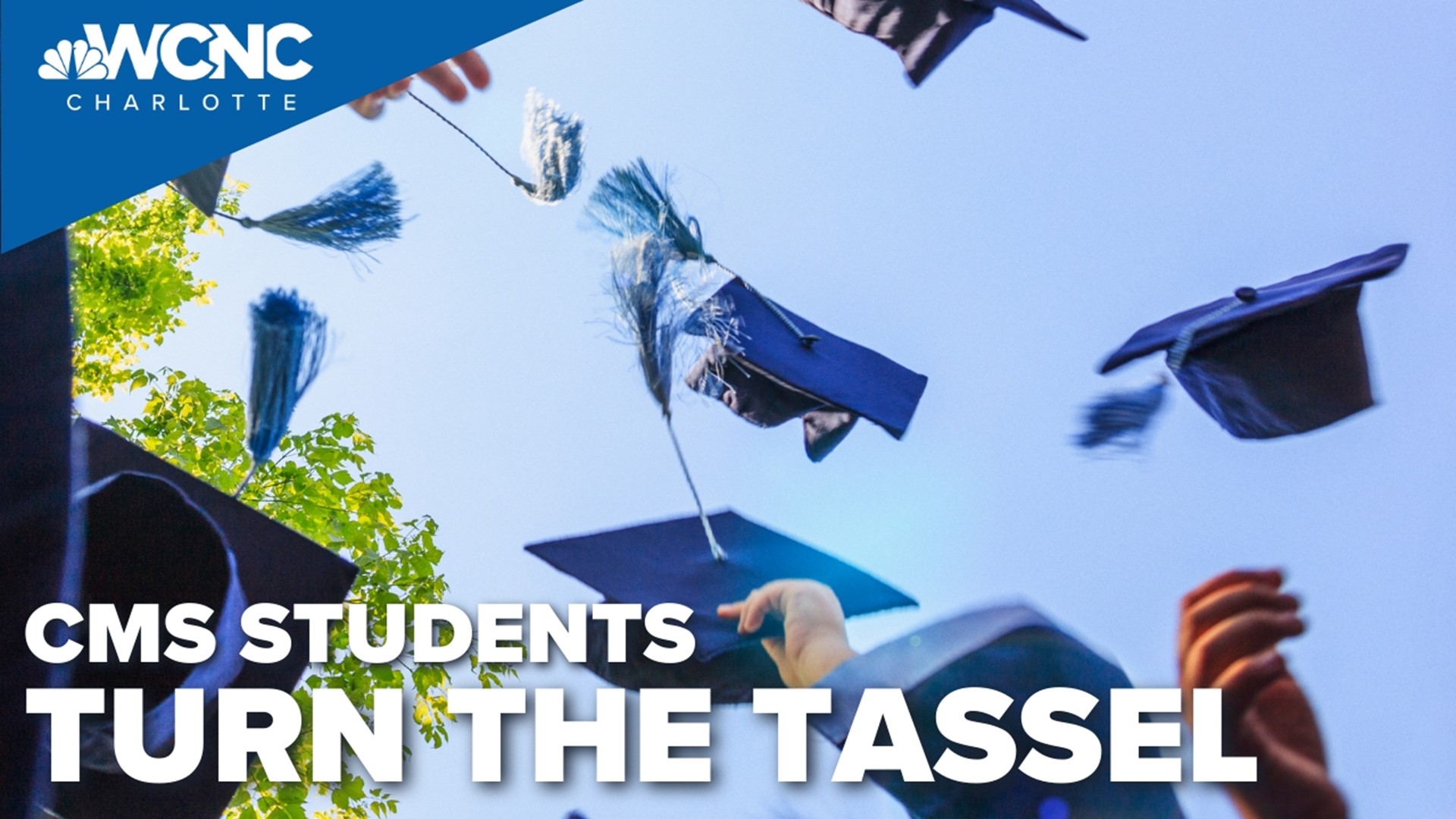The image is a celebratory poster for an upcoming graduation set against a beautiful, clear blue sky. In the top left corner, the WCNC Charlotte logo is prominently displayed, featuring the NBC emblem. Several blue graduation caps with matching tassels are caught mid-air, indicating the joyous moment of students tossing their caps. The caps are thrown by a diverse group of students, as indicated by a range of hand colors visible at the bottom of the image. A couple of trees can be seen on the left side, adding to the outdoor setting. Bold white text at the bottom of the poster reads, "CMS students, turn the tassel," emphasizing the significant milestone. There are no dates or additional information included, suggesting it is a general announcement for the upcoming graduation season.